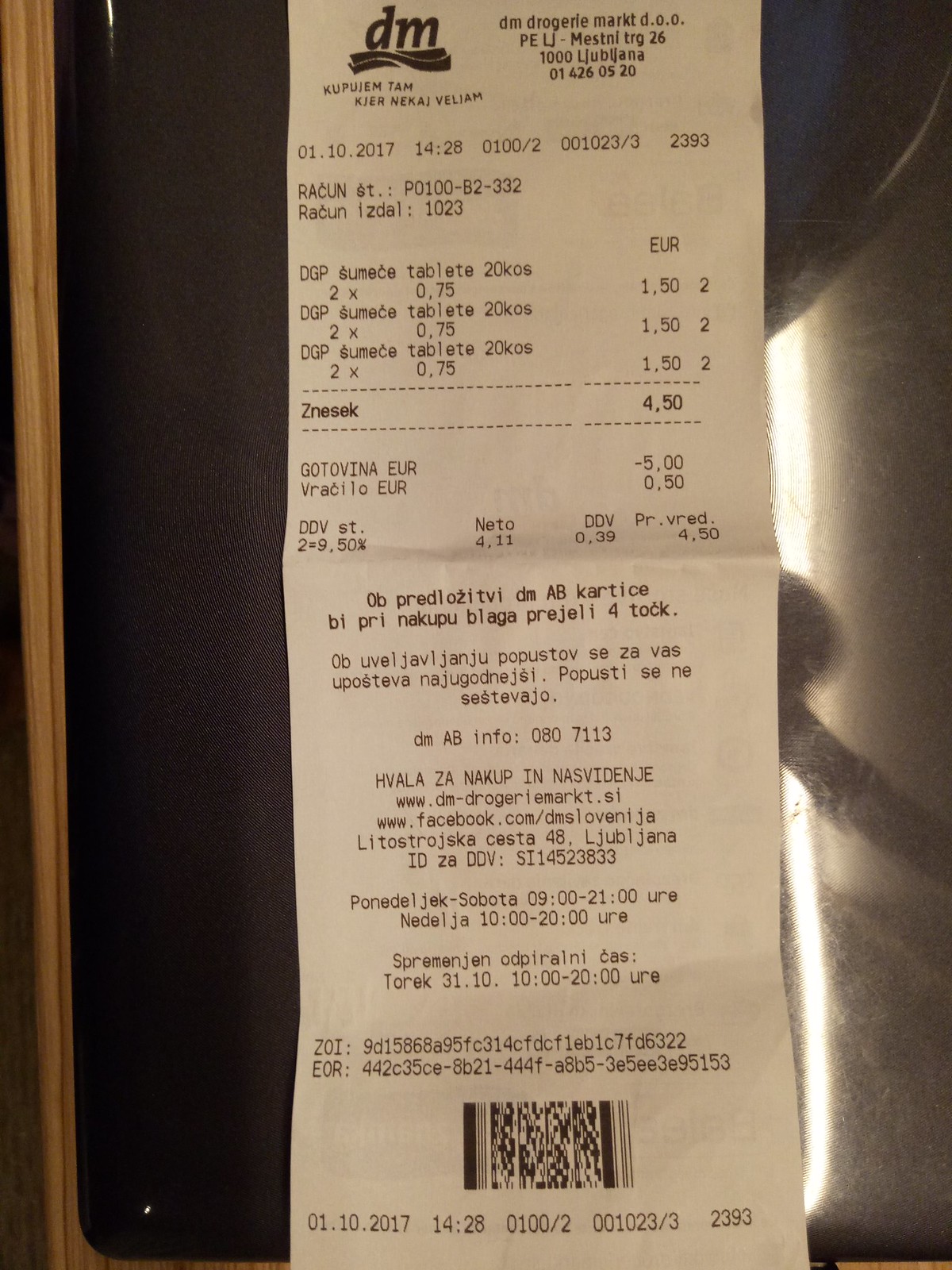This is a detailed photograph in portrait format showcasing a white paper receipt on a reflective black glass-like surface with a wooden frame, reminiscent of a picture frame. The store logo at the top features the letters "DM" with wavy black lines underneath, indicating it's from DM Drogerie Market in Ljubljana. An address is visible to the right of the logo and a store name in a non-English language follows below. The date on the receipt is 01.10.2017, with the time stamped as 14:28. Sequential numbers, possibly denoting register and store details, are listed as "0100/2", "001023/3", and "2393." 

The receipt features items labeled as "DGP", "SUMUCE", and "TAVLETE," likely some form of tablets, each priced at €0.75 and listed with a quantity of 2, totaling €1.50 per line and an overall sum of €4.50. The total amount is confirmed under the label "ZN-ESEK," with a cash payment noted as "GOTOVINA EUR," resulting in a change of €0.50 from a €5 payment. Various additional numbers and codes, including "DDV ST 29.50%", are printed, potentially indicating tax or discount details. At the bottom, a barcode is present for scanning.